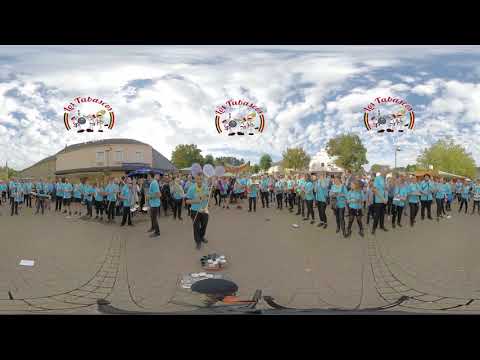This photograph captures an outdoor event with a panoramic and fisheye effect, creating slight distortion in the image. A large group of around 40 to 50 people, dressed uniformly in light blue shirts and black pants, are gathered primarily in the center and extend outward in a formation reminiscent of a V or a zigzag. It appears they might be a marching band or a similar group of performers, as some members are holding musical instruments like a tuba. They are standing on a brownish-red brick or tiled road, surrounded by various structures and natural elements.

To the left of the group stands a tall, gray building with an arched roof, perhaps a concert hall, while to the right, there are some white and tan buildings scattered amidst random trees. Above them, the sky is vibrant blue with puffy white clouds, giving a serene backdrop to the bustling scene below. Adding to the festive atmosphere, three circular logos featuring arched text and cartoonish images of a band float above the crowd, further emphasizing the theme of the event. Thin black bars frame the top and bottom of the image, enhancing the panoramic effect and contributing to the overall composition of the photograph.